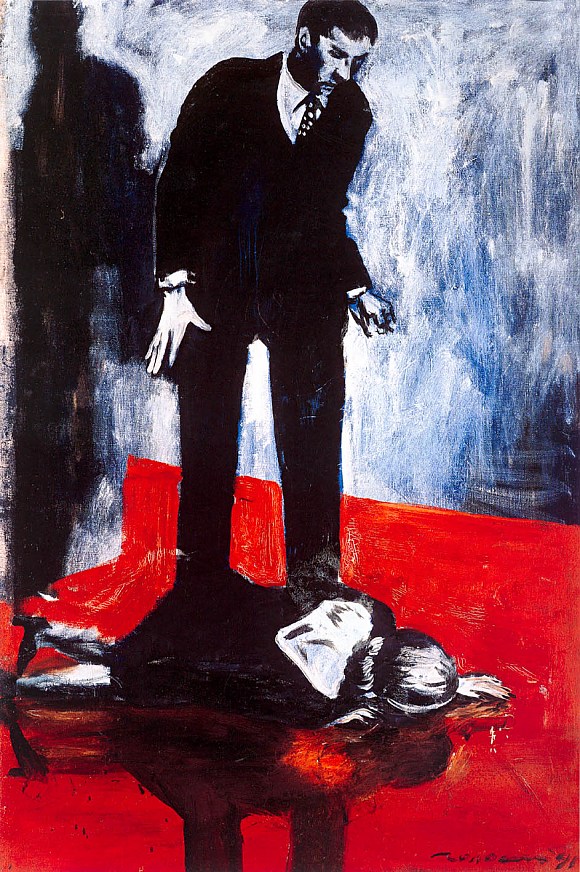The image depicts a striking and detailed painting of a man standing over a woman lying face down on a red floor. The male figure, dressed in a black suit, white shirt, and a black-and-white polka-dotted tie, casts a dark shadow that extends across the body of the woman. His expression of surprise or guilt is evident as he looks down at her. The woman's hair is tied in a ponytail, and she is wearing a v-neck dress that exposes her back, with a scarf around her neck. Both the man's legs and a dark reflection of the woman can be seen on the floor. The room is characterized by its black and white walls with hints of blue, painted with highly textured brushstrokes that create a haunting, shadowy atmosphere. The artist's name is inscribed at the bottom right corner of the painting.